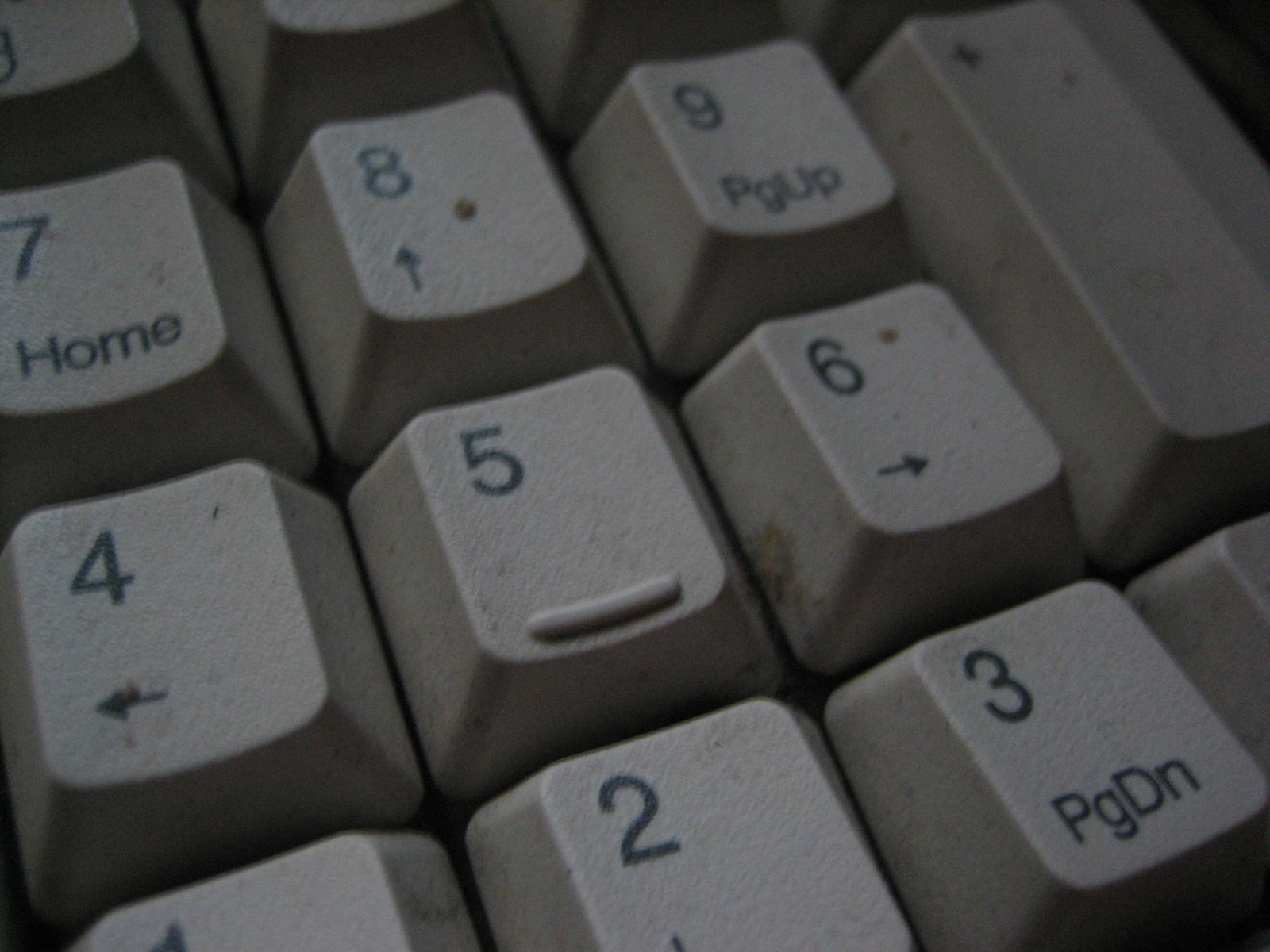The image is a close-up photograph of a well-used numeric keypad on an off-white or light gray keyboard, likely from a dated desktop PC. The keypad is tilted slightly with the numbers slanting upwards to the right. Visible keys include 7, 8, and 9 at the top, with 4, 5, and 6 in the middle, and, partially at the bottom, the numbers 1, 2, and 3. A plus symbol key is in the upper right corner. The keypad includes several function keys: the 9 key also has "PG up," the 7 key has "home," the 8 key has an up arrow, the 4 and 6 keys have left and right arrows, and the 3 key has "PG DN." The 5 key features a tactile bump for orientation. The photograph is dimly lit, highlighting the dirt, grime, and possible liquid stains scattered across the keypad, enhancing the keypad's aged and grimy appearance.